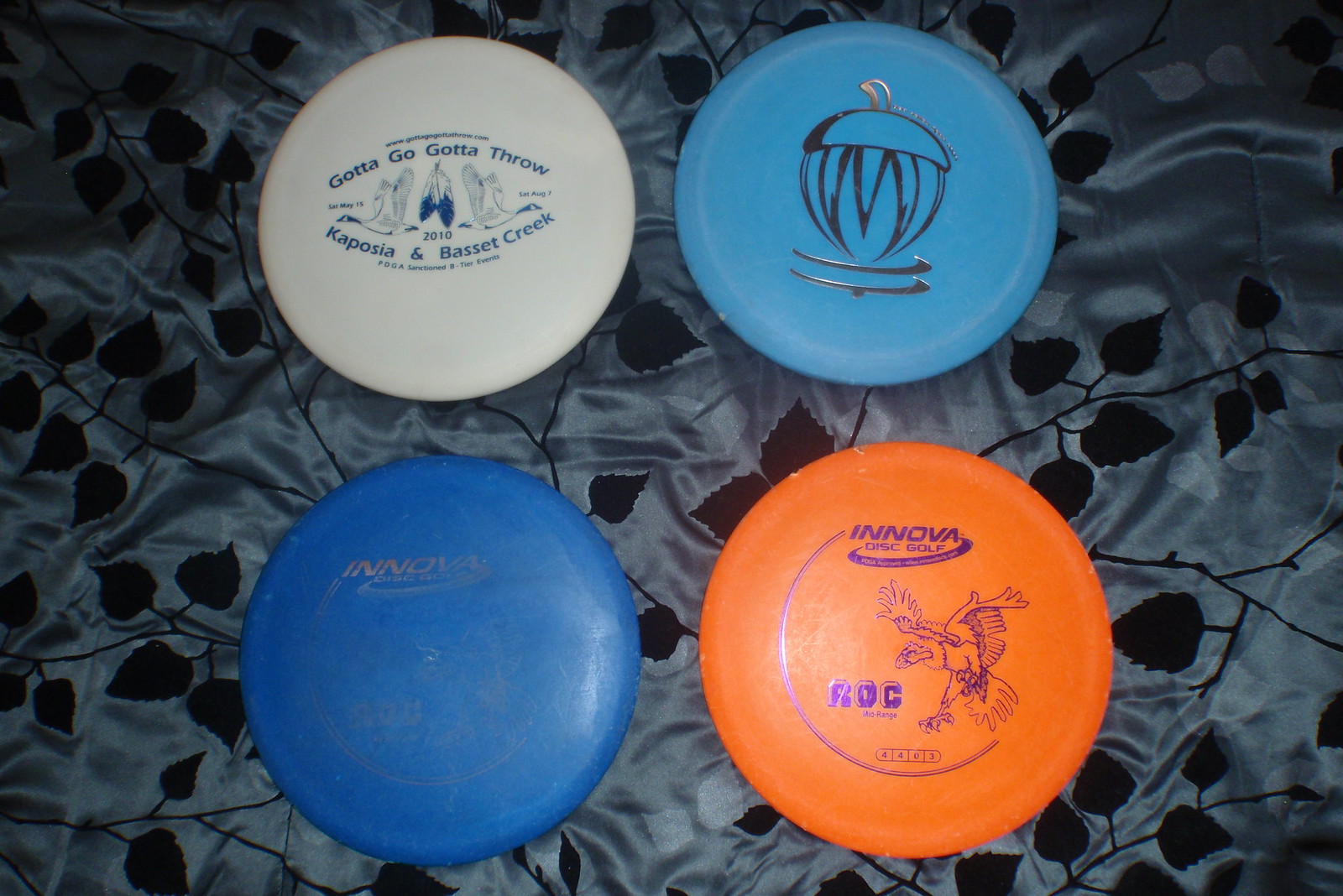The image features a detailed arrangement of four well-used frisbee discs displayed on a dark grey silk bedsheet adorned with black leaf patterns. The photograph is landscape-oriented, capturing the frisbees laid out in a neat 2x2 grid, making them the focal point of the composition. 

The top left frisbee is white with black text that reads "Gotta Go, Gotta Throw, Kaposia and Bassett Creek 2010." To its right is a light blue frisbee, adorned with an image of what appears to be a gold-colored acorn or stylized apple with elongated fangs and black swishes. The bottom left frisbee is dark blue with faded gold text that says "Innova," indicating signs of wear. Finally, the bottom right frisbee is a vibrant neon orange, also branded "Innova" in blue letters with a swirling design, featuring a purple-outlined bird and the text "ROC" next to it.

The backdrop and careful arrangement suggest the frisbees might be photographed for an online listing, such as eBay, where their condition and design details are clearly showcased for potential buyers.